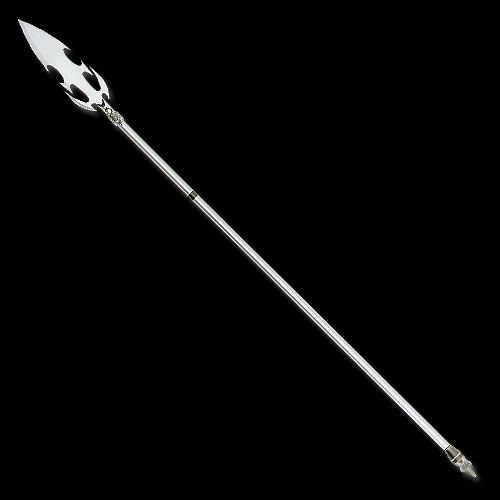The image features a strikingly detailed white dagger set against a solid black background. The dagger, oriented from the bottom right to the top left, showcases a meticulously designed blade that tapers to a pointed arrowhead at its tip. The blade then narrows before expanding into two additional points on each side and tapering again near the hilt in a pattern of alternating curves and points. 

The dagger's handle, constructed of silver with a shiny, metallic finish, appears slender and elongated. About a quarter of the way down the handle, a distinctive black strip encircles it. At the base of the handle, a black section with ornate detailing and possible embellishments such as jewels or metal balls enhances its appearance.

Overall, the composition of the image emphasizes the stark contrast between the black background and the luminous silver and white of the dagger, highlighting its intricate design and creating a visually compelling scene.